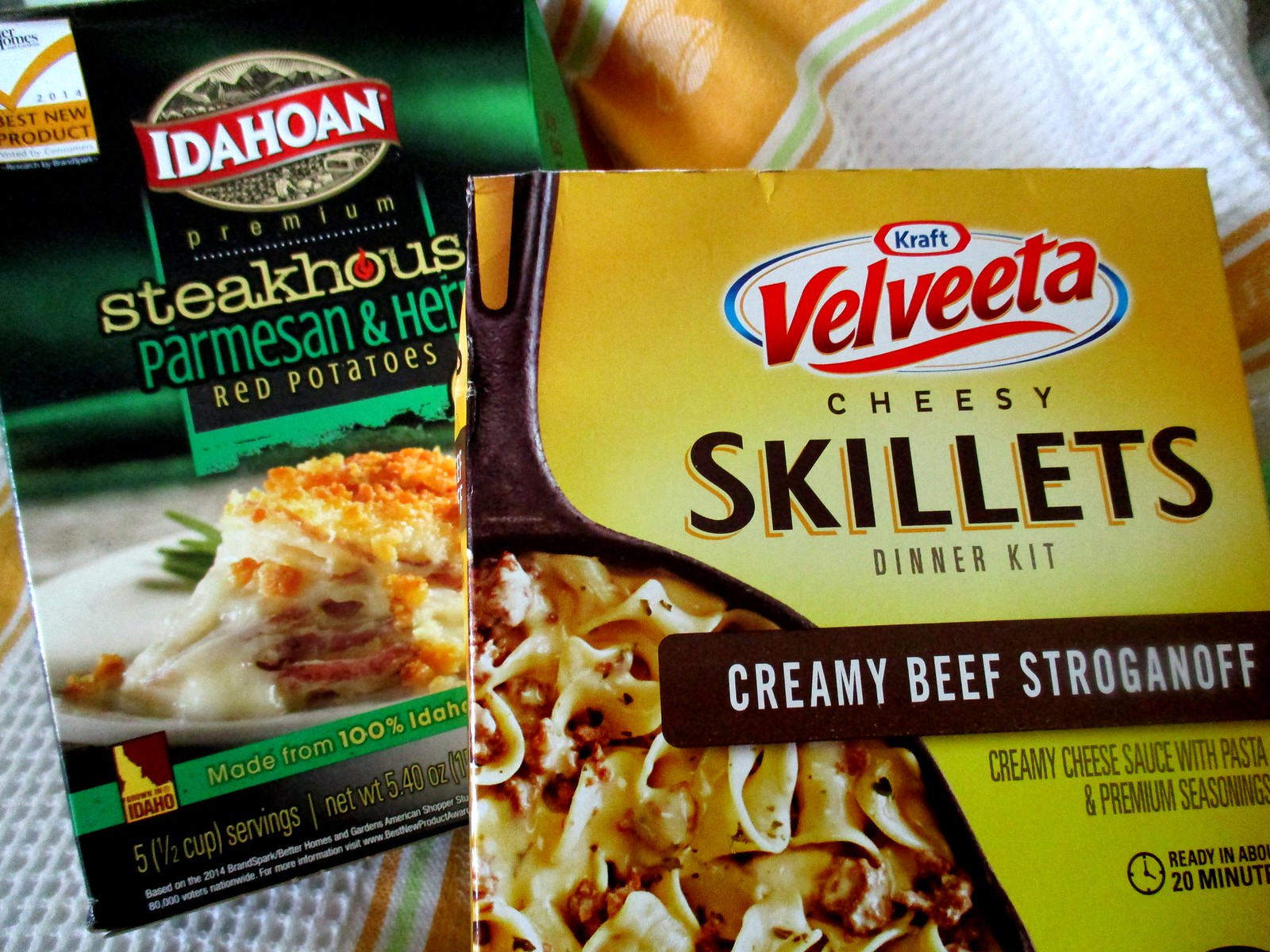This is a close-up photograph of two food packages placed on a white kitchen towel with an orange border showcasing teacups. In the foreground on the right is a predominantly yellow box of Kraft Velveeta Cheesy Skillets Dinner Kit, specifically the Creamy Beef Stroganoff variety. The packaging features the Velveeta logo in red with details indicating it's a creamy cheese sauce with pasta and premium seasonings, ready in about 20 minutes. There is an image of the creamy beef stroganoff served in a cast-iron skillet at the bottom left of the box. To the left and slightly behind it is a predominantly green package of Idahoan Premium Steakhouse Parmesan and Herb Red Potatoes. The box information highlights that it is made from 100% Idaho potatoes and offers five half-cup servings, with a net weight of 5.40 ounces. The package also displays an image of the parmesan and herb red potatoes on a plate, emphasizing its gourmet appeal.